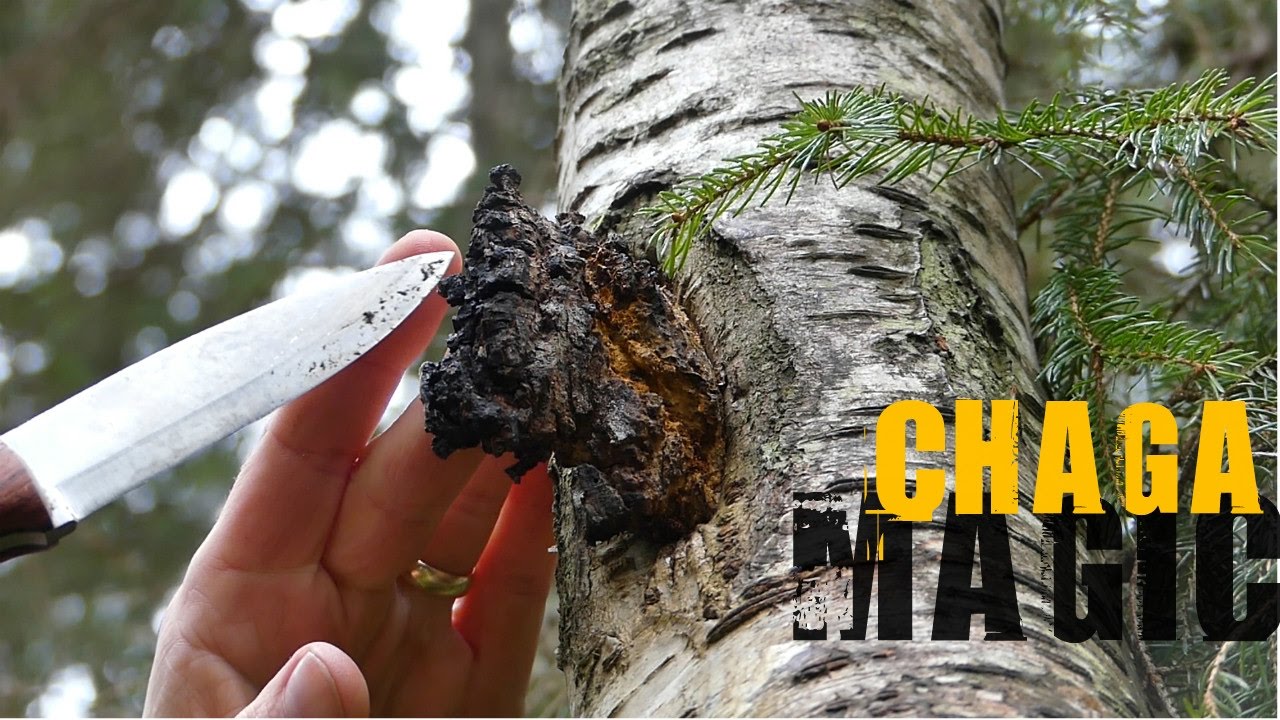The image is a close-up of a pine tree trunk with light grayish bark. A dark brown and black irregular growth or stub protrudes from the tree. A hand with a gold wedding ring is holding a knife that is aimed at this growth, presumably to cut or scrape it off. The knife has visible residue, indicating prior contact with the growth. The background consists of blurred leaves and possibly other trees, further emphasizing the rugged, outdoor setting. Overlaying the photo, in large rugged-themed fonts, are the words "Chaga Magic," with "Chaga" in orange and "Magic" in black, located at the bottom right of the image.